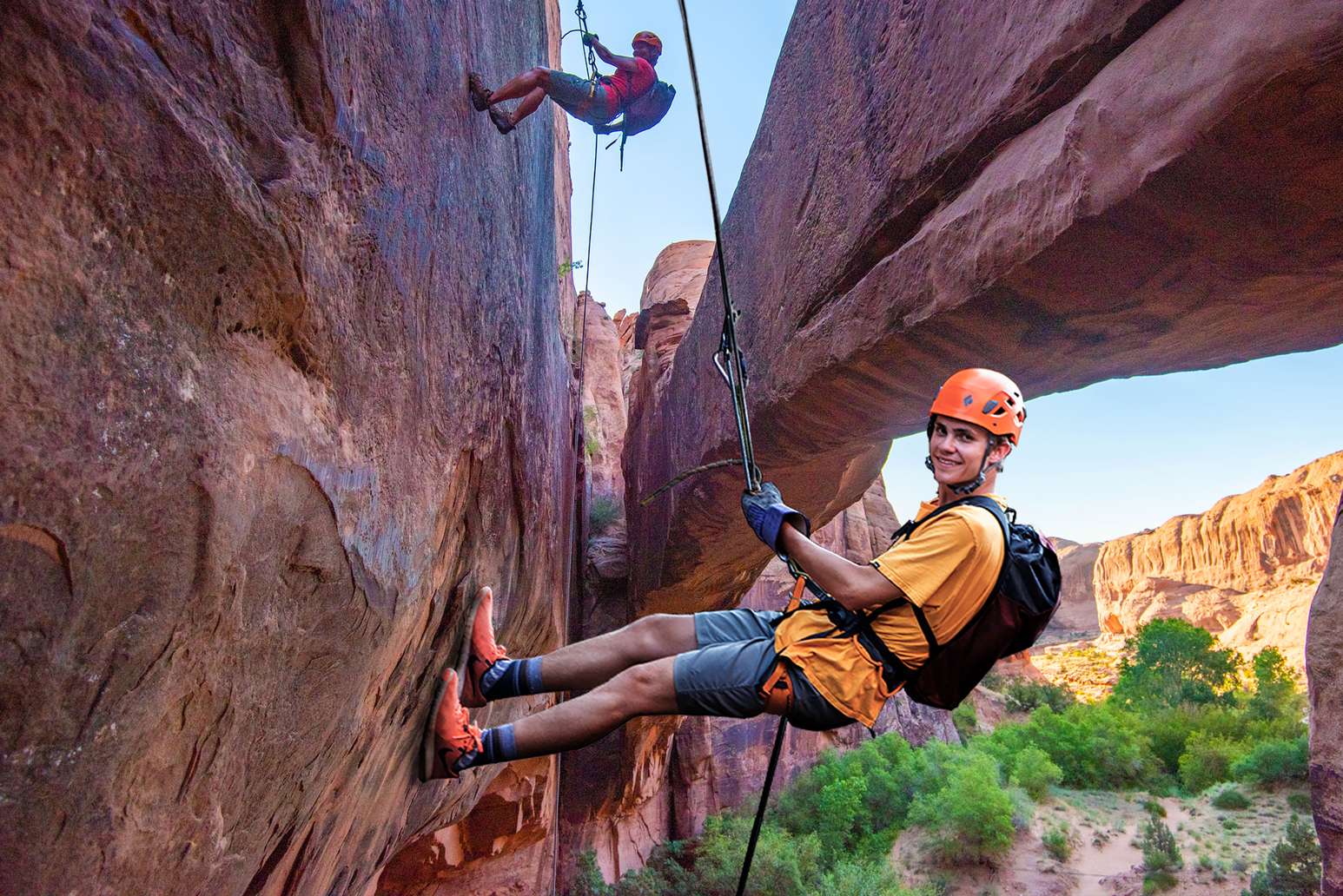The photo captures an exhilarating moment of two rock climbers amidst the stunning landscape reminiscent of Utah. Dominating the center is a male climber in a yellowish-orange shirt and bluish shorts, highlighted against the rugged terrain with his orange helmet and shoes. He is horizontally positioned, with his legs pointing left and body to the right, suggesting he is rappelling down. His left hand firmly grips a rope that extends out of view, adding to the dynamic feeling of descent. He also sports a black backpack and looks directly at the camera with determination. Above him, another climber, dressed in red with a matching helmet and shorts, is visible at the top of the photo, also engaging in rappelling. The climbers are framed beautifully against a vivid blue sky, with dark reddish-brown rocks and natural arches forming a dramatic backdrop. The scene is further enriched by green trees and an orange rocky hillside at the bottom right, providing a contrast to the rocky corridor the climbers navigate. This image vividly portrays the adventurous spirits of the climbers against the majestic and expansive outdoor setting, clear and crisp in detail.